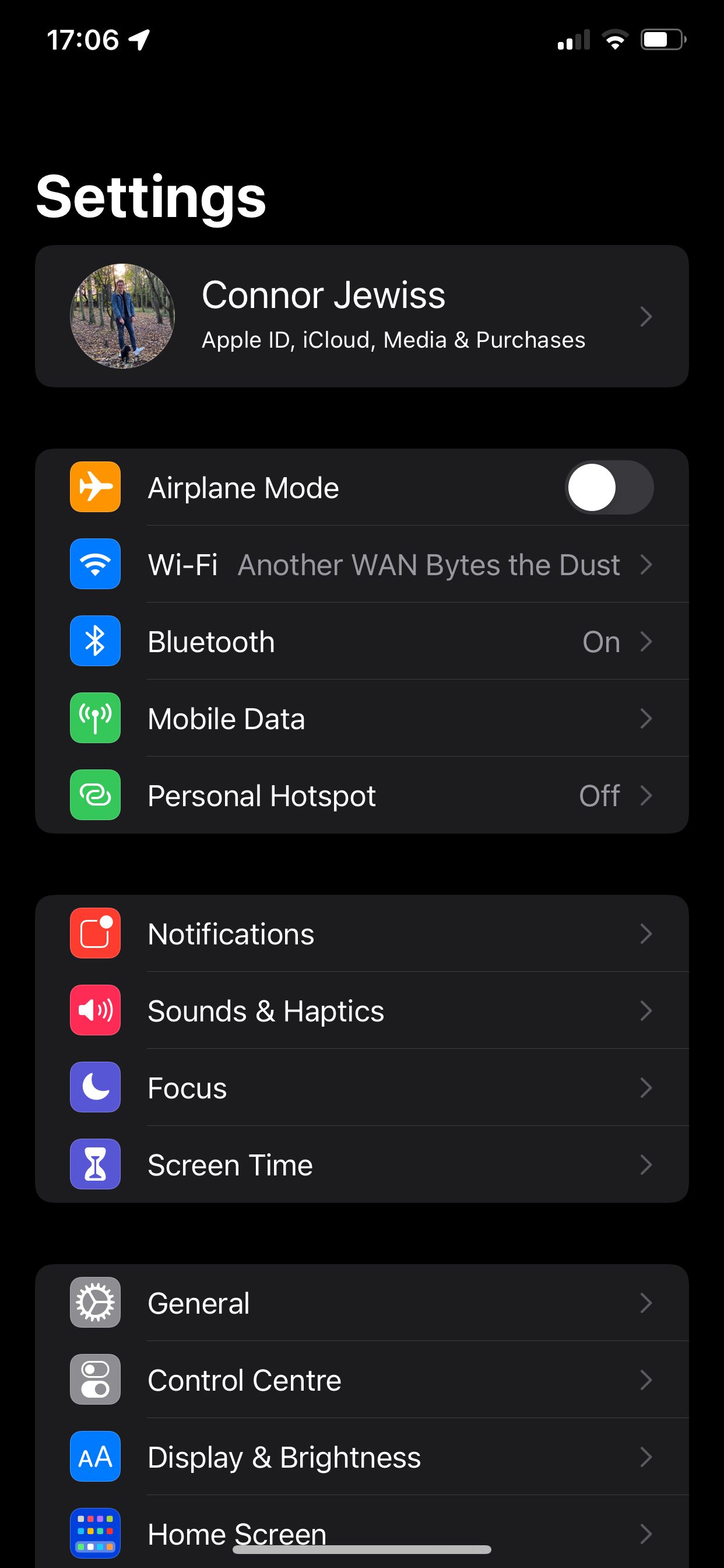This screenshot from a cell phone displays a black background with the time "17:06" at the top center in white text. To the right of the time, the icons for cell signal, Wi-Fi signal, and battery percentage are neatly aligned. Below the status bar, white bold text with a capital 'S' reads "Settings."

Underneath "Settings," there is a tab that reads "Connor Jewis, Apple ID, iCloud, Media & Purchases," wherein "Connor" is spelled C-O-N-N-O-R with a capital C, and "Jewis" is spelled J-E-W-I-S-S with a capital J. Adjacent to this text on the left is a small circular icon containing an image.

Moving further down, the list of settings options begins with "Airplane Mode" indicated as turned off, followed by "Wi-Fi" and an additional label "WAN," which might be a network name. Next, "Bluetooth" is shown as on, while "Mobile Data" and "Personal Hotspot" are listed with the latter being off.

The settings list continues with sections labeled: "Notifications," "Sounds & Haptics," "Focus," and "Screen Time." Further down, additional categories are displayed including "General," "Control Center," "Display & Brightness," and "Home Screen."

Each section or setting option is accompanied by a small square icon containing a graphic on the left and a right-facing arrow on the right, to indicate further navigation. At the very bottom of the screen, there is a faint grey line with an arrow to the right, providing a visual cue for additional options beyond the visible menu.